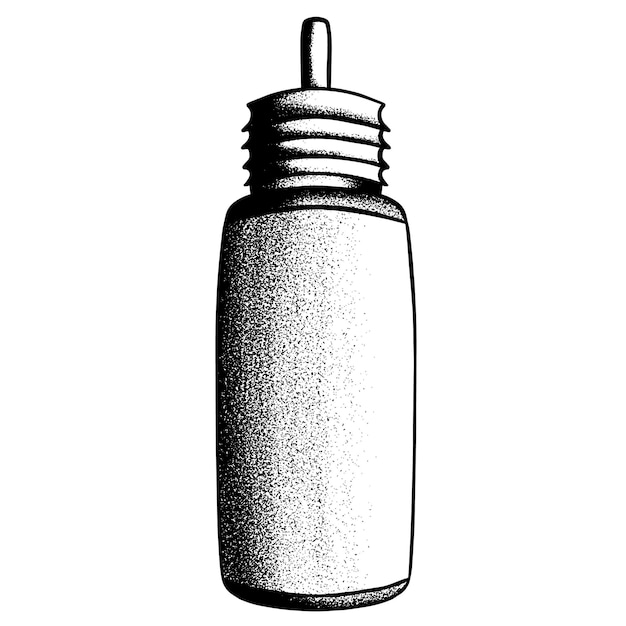This detailed black and white drawing, possibly created with ink or pen, depicts a salt container against a stark white background. The cylindrical bottle-like structure has a tall, slender form with varying shades of black for shading and detailing. The bottom section is darker, transitioning to a predominantly white upper body with scattered black speckles on the left side, indicating it's full of salt granules. The container is topped with a ridged, screw-top circular lid that extends upwards with three to four visible bands. Above these ridges, the lid culminates in a small dowel-like extension or straw, adding a functional element to the design. The contrast between the black and white shading intensifies the visual depth and highlights the detailed texture of the container.